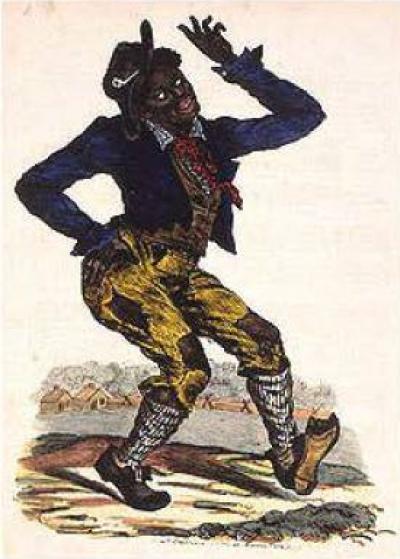In this old, vintage drawing, an African American man is depicted dancing with his body contorted in a dynamic and expressive pose. He is looking skyward with his mouth slightly open, his left hand raised above his face, and his right hand placed firmly on his hip. He is sticking his butt out while his left foot kicks off a worn shoe, and he steps energetically on a dirt road. The man is dressed in tattered, mismatched clothes that resemble rags; he wears a dark blue, almost purple, or navy jacket, a vest, a loose tie, and a checkered shirt. His yellow pants, patched with brown fabric, and long socks contribute to his worn appearance, along with his Civil War-era hat. His four-fingered hand adds a unique detail to his character. The background features rustic, old houses, giving a glimpse of a distant village under a worn, pinkish sky. The scene captures a lively moment filled with historical and cultural significance.